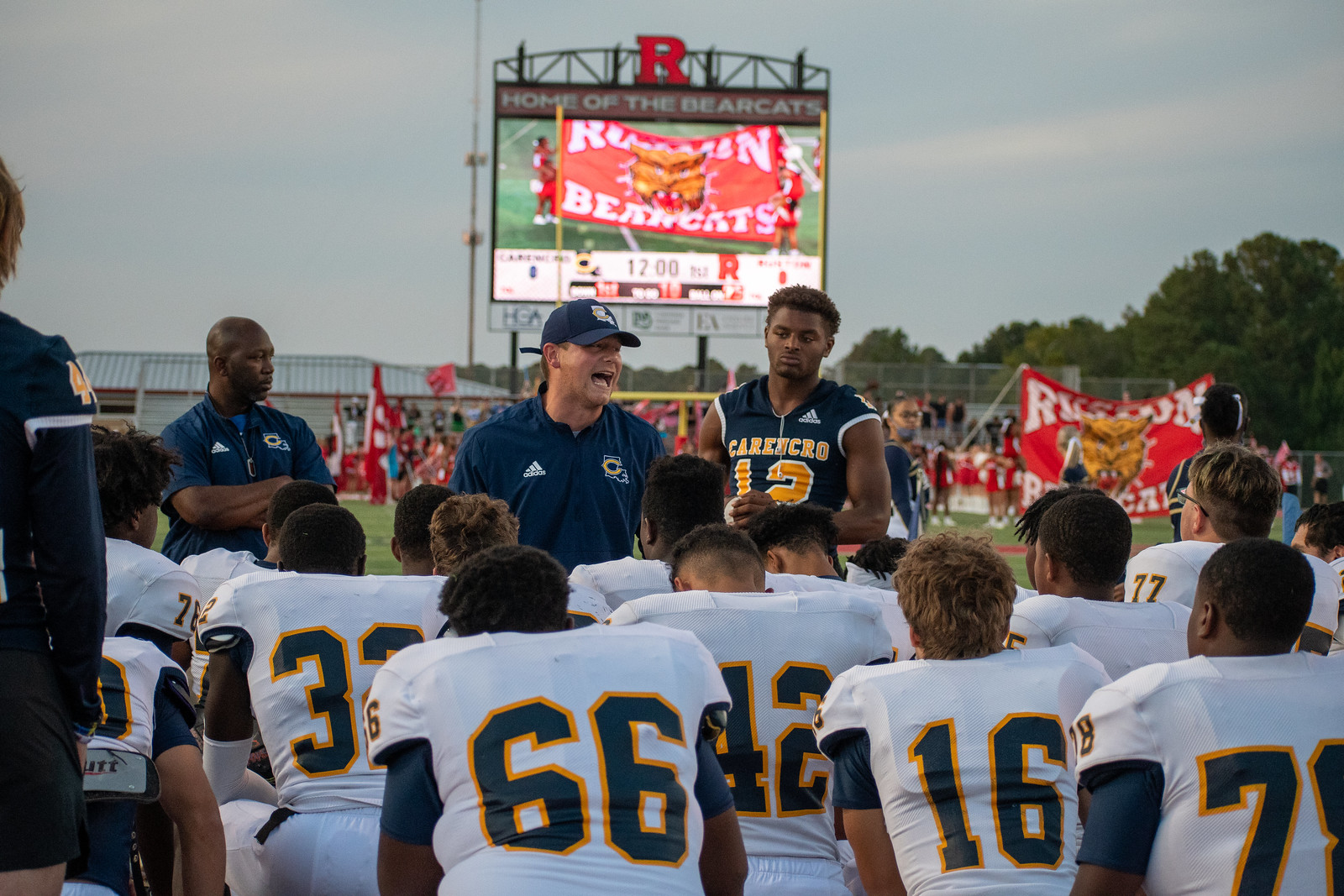In this detailed sunset photo taken at a football field, a group of football players in white jerseys with blue and yellow numbering huddle together with their backs to the camera. Among the visible numbers are 66, 16, and 42. The players' focus is on their coach, a white male in a blue polo shirt and matching baseball cap, who stands in front of them, delivering a pep talk. To the coach's left stands another man, a black male, also in a blue polo shirt, while on the right, a black football player in a blue sleeveless jersey marked with "Carregro" and the number 12, listens attentively. The scene unfolds in the vibrant atmosphere of a football stadium, with cheerleaders, fans, and red and white flags in the background. Dominating the distance is a large teleprompter screen that reads "Home of the Bearcats," which displays live footage of the game and team spirit. The picturesque ambiance is enhanced by trees framing the field and a darkening sky, suggesting that the image was captured at sunset.